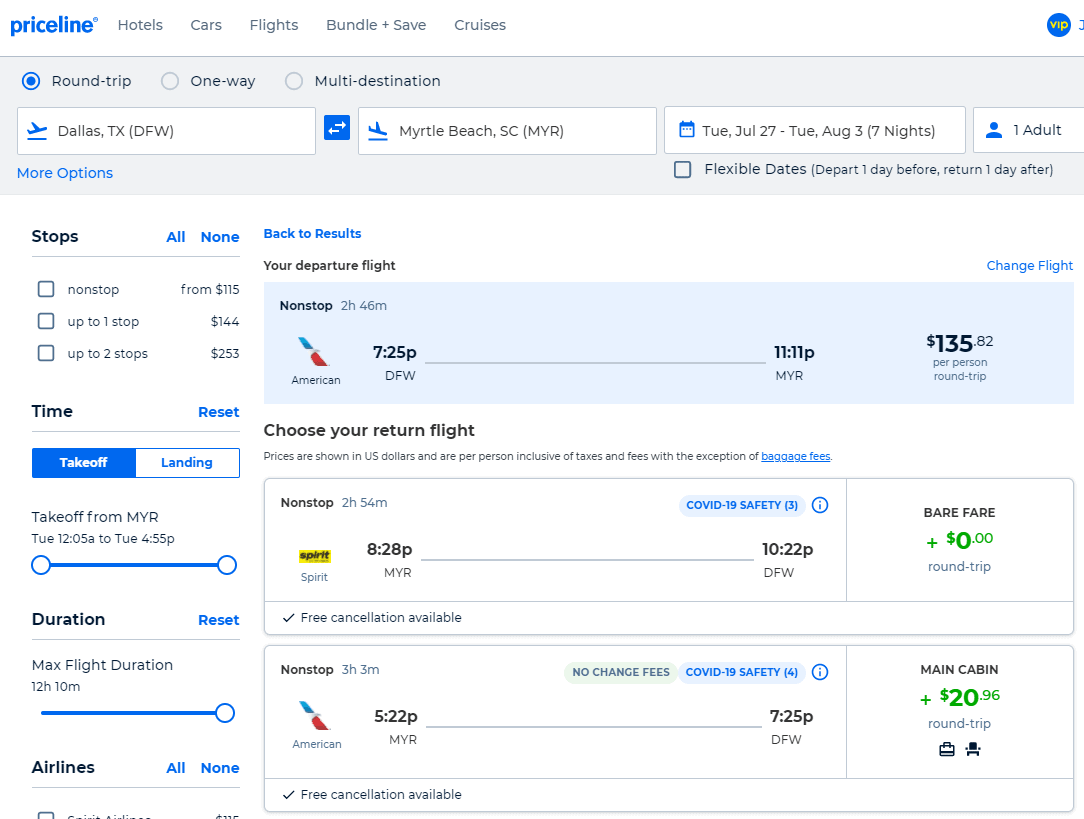The web page from Priceline showcases a detailed flight search interface, designed with user-friendly interactive elements for booking a trip. 

In the top-left corner, the Priceline logo in full blue stands out, accompanied by a navigation menu with clickable buttons: "Hotels" (in gray), "Cars," "Flights," "Bundle + Save," and "Cruises." Below this, there is a dark gray rectangle highlighting the selected "Round Trip" option, marked by a blue dot encircled by another blue dot. A blue airplane icon lifting off from a blue line indicates a flight departing from Dallas, TX (DFW), with "Dallas, TX (DFW)" displayed in black text.

Adjacent to this information, a square icon featuring bidirectional arrows allows users to switch between the origin and destination. Below, a clickable "More Options" link in cyan blue offers additional choices. The destination is Myrtle Beach, SC (MYR), denoted by an icon of a plane landing on a line. The text "Myrtle Beach, SC (MYR)" is in black.

A rectangle follows, showing the travel dates: "Tuesday, Jul 27th - Tuesday, Aug 3rd (7 nights)" with a blue calendar icon. To the right of this, a silhouette icon informs that the booking is for "1 Adult."

Beneath the search criteria, a dropdown on the left allows users to filter stops with options "All" or "None" in bold blue, while a "Back to Results" button appears on the right. One flight option shows a "Non-stop" flight with the American Airlines logo—a stylized eagle with blue and red wings. The flight details are "7:25 PM (DFW) – 11:11 PM (MYR)" at a price of "$135.82 per person, round-trip." 

Additional information includes a prompt to "Choose Your Return Flight." Prices are shown in US dollars per person, inclusive of tax and fees, with an exception noted for "baggage fees" in clickable blue text. 

The first return flight detail reads "Non-stop," lasting "2h 52m," offered by Spirit Airlines (displayed in a yellow box with black text). The flight times are "8:28 PM (MYR) – 10:22 PM (DFW)." A COVID-19 safety notice is prominently displayed in a cyan blue oval, with a circled 'i' for further information.

The fare details include a "Bare Fare" option, specified as "$0.00" in green, and another American Airlines flight listed at "5:22 PM (MYR) – 9:25 PM (DFW)." A marking "Free Cancellation Available" is included, along with tags for "No Change Fees" in light green and blue, and "Main Cabin" with an additional cost of "$20.96," along with icons representing amenities like baggage and seating.

This meticulously designed web page offers comprehensive options for booking a round-trip flight, providing thorough details to ensure an informed and hassle-free booking experience.